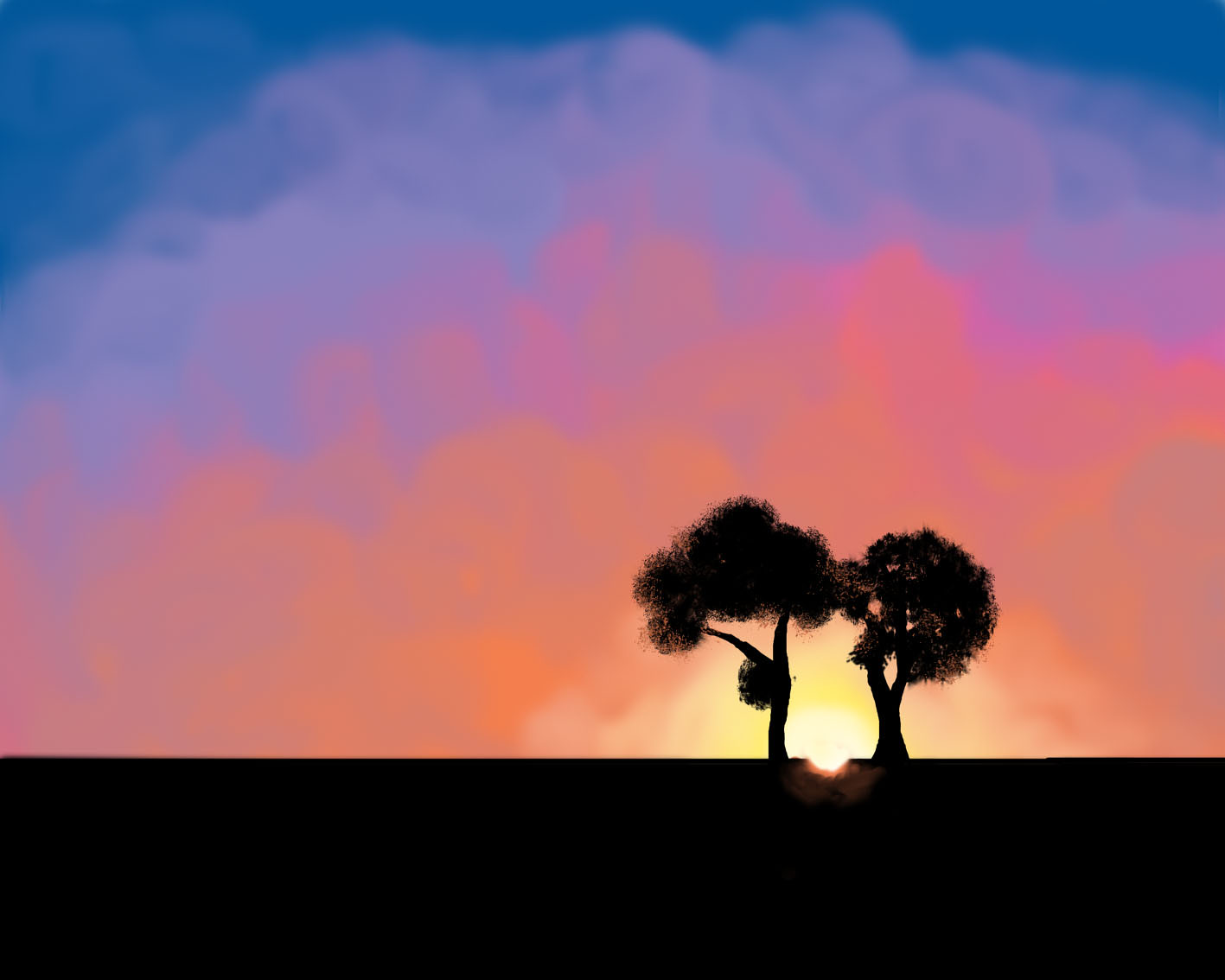This image captures a stunning hand-painted sunset, though the techniques used leave some ambiguity between traditional painting and digital artistry. The sky transitions through a breathtaking palette: starting from a rich dark indigo at the top, it fades into vibrant violet, fuchsia, and shades of orange, finally lightening into yellow around the sun. Fluffy, semi-transparent white clouds float across the top left, blending delicately with the underlying hues. 

Near the horizon, the sun sits as a bright semi-circle, partially dipping into the dark land below, which is represented by a stark black line stretching across the bottom quarter of the image. Positioned center-right, the sun illuminates the scene with a warm glow. 

On either side of the sun, two silhouetted trees stand sentinel. The tree to the right has a thicker trunk with blotches of leaves, while the one on the left has a thinner trunk that splits into two main branches. Both trees are depicted with expressive, almost haphazard brushstrokes, contributing to a sense of texture and realism in their leaf canopies. The overall composition is devoid of any signatures or wording, allowing the viewer to fully immerse in the painted twilight landscape.